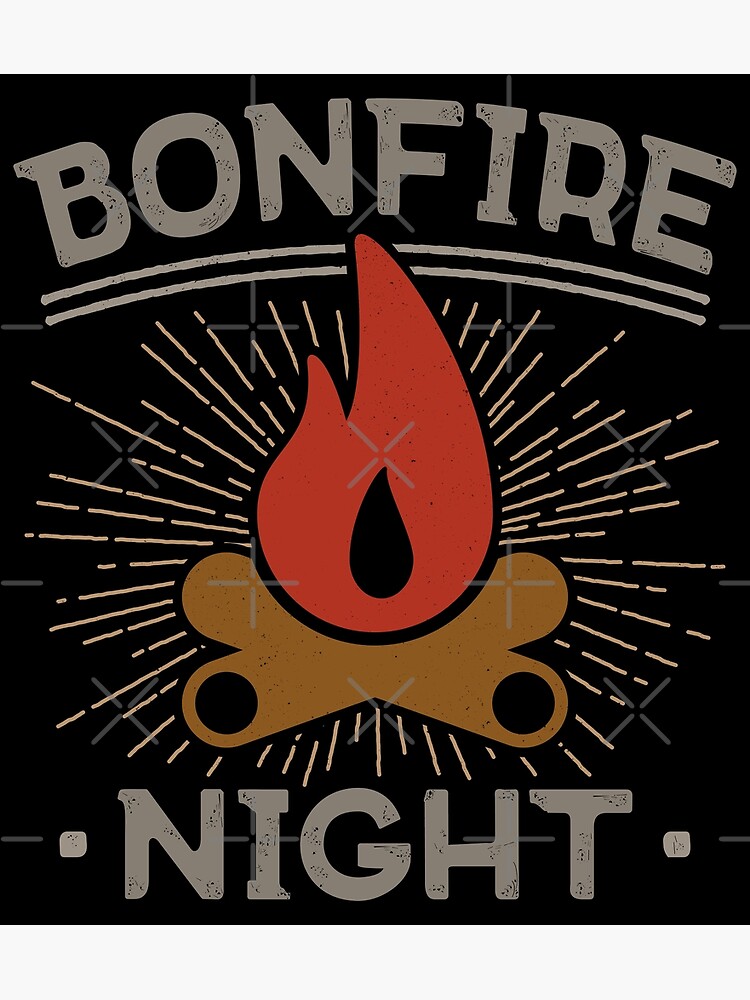This detailed poster showcases an inviting "Bonfire Night" theme with a central illustration of a bonfire. Two brown wooden logs are depicted crisscrossing at the base, with vibrant red and orange flames rising above them. Radiating from the bonfire are thin white lines, suggesting either radiant heat or glowing light. At the top of the poster, the words "BONFIRE" are prominently displayed in an arched, gray all-caps font, accompanied by a double underline. At the bottom, the word "NIGHT" is also in gray, all caps but in a straight line, flanked by bullet points on either side. The entire image is set against a solid black background with faint, cross-shaped watermarks scattered throughout, adding a subtle texture. This minimalistic yet striking design communicates the essence of a community bonfire event without additional details.